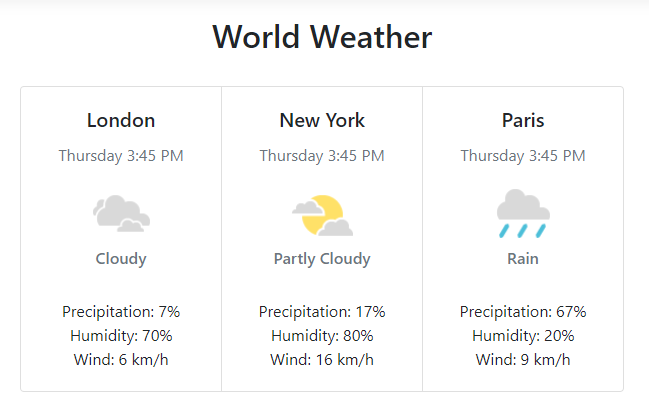The image is a screenshot of a weather app interface featuring the weather conditions for three cities: London, New York, and Paris. 

At the top, the app displays a white header area with a thin gray line at the very top, followed by the title "World Weather" in black text. Below the header, the weather information is segmented into three adjacent rectangles, each representing a different city and its weather details.

1. **London**:
    - **Date & Time**: Thursday, 3:45 PM
    - **Weather Condition**: Cloudy, represented by a cloud icon
    - **Details**:
      - Precipitation: 7%
      - Humidity: 70%
      - Wind: 6 km/h

2. **New York**:
    - **Date & Time**: Thursday, 3:45 PM
    - **Weather Condition**: Partly Cloudy, depicted with a sun partially covered by a cloud in the upper left corner and another cloud in the bottom right corner
    - **Details**:
      - Precipitation: 17%
      - Humidity: 80%
      - Wind: 16 km/h

3. **Paris**:
    - **Date & Time**: Thursday, 3:45 PM
    - **Weather Condition**: Rain, symbolized by a cloud with three blue raindrops
    - **Details**:
      - Precipitation: 67%
      - Humidity: 20%
      - Wind: 9 km/h
    
Below the rectangles, there is a blank white space devoid of any further content.